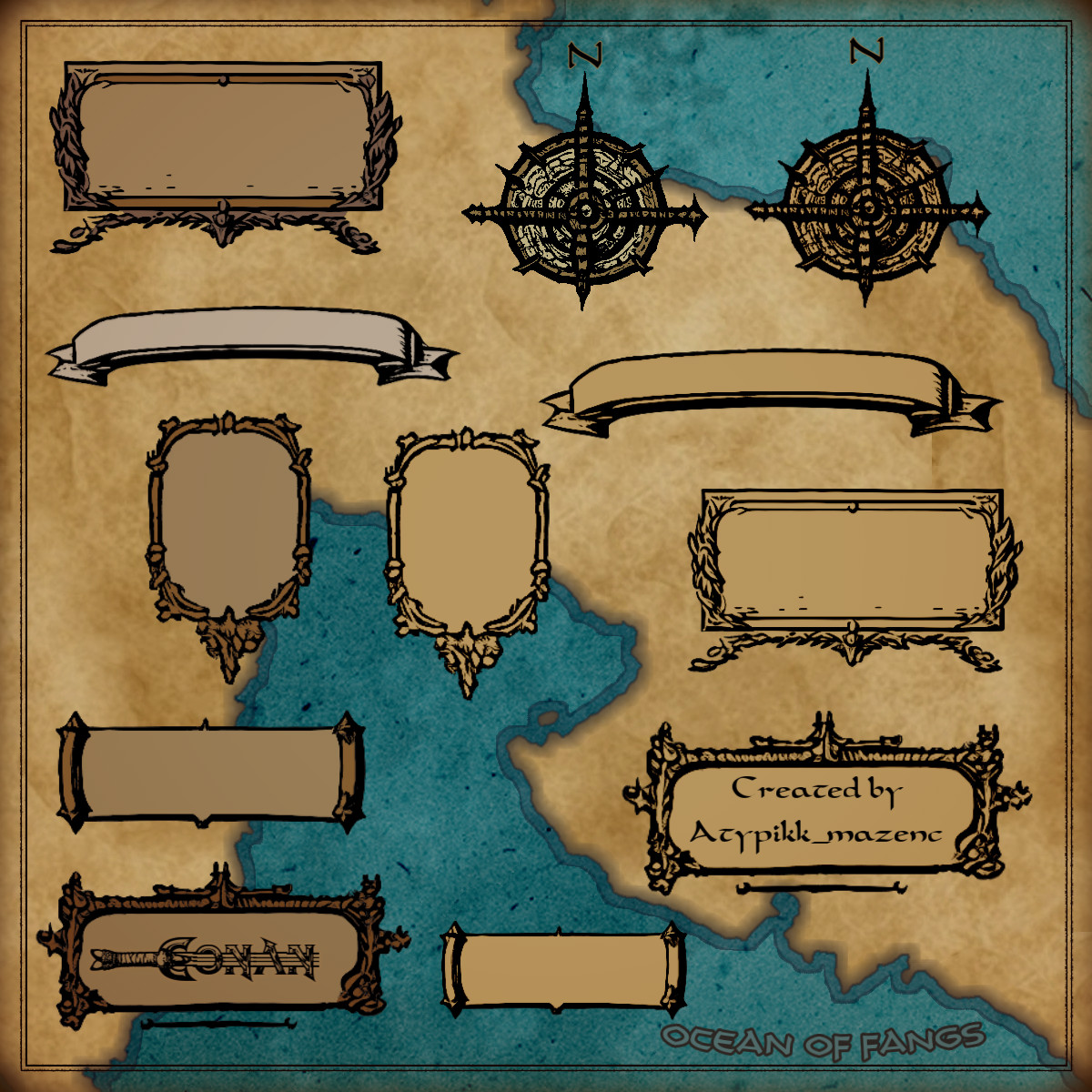The image depicts a detailed, hand-drawn, cartographic map that resembles elements from a video game interface. The map showcases a landmass with intricate borders, taking on a horseshoe shape, with brown representing the land and blue for the water. The landmass stretches from the lower left to the top right before looping down towards the right. In the southern central portion and the northwestern corner, water bodies are labeled "Ocean of Fangs."

Scattered across the map are various ornate headers and labels, primarily blank, designed to hold information. These labels have a curl design, giving the map a historic or fantasy feel. Two of these panels contain specific details: one in the bottom right corner displays the text "Created by AZYPKK Mazine" in a decorative script, and another in the lower left corner features a graphic of a sword with the name "Conan" seemingly pierced by the sword. Additionally, the top right corner of the map features two compass roses, one in a pale color and another in deep wood tones, both marked with an 'N' to indicate north.